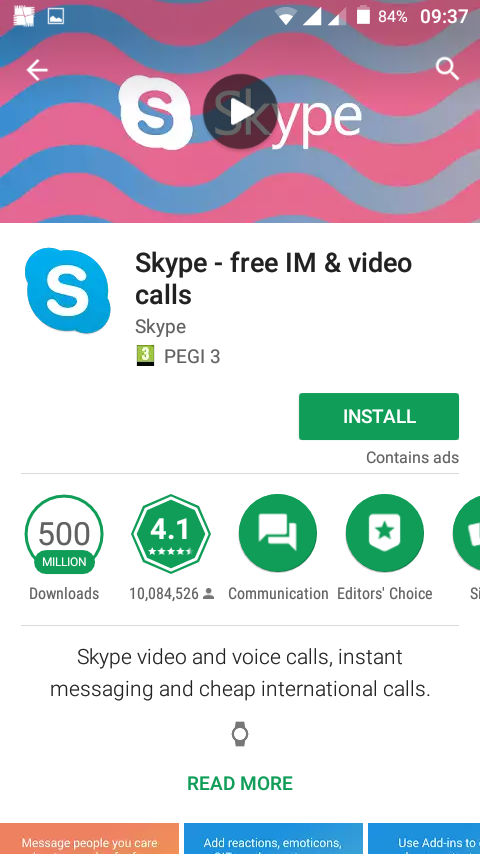This is a detailed screenshot captured on a mobile phone displaying the Skype section in the Play Store or App Store. 

At the top of the screen, various status icons are visible: a Windows icon, the Gallery icon, and the Wi-Fi icon, which is half full. To the right, two mobile data icons are shown, one full and the other half-full, followed by the battery icon indicating 84 percent charge. The time displayed on the phone is 9:37.

Below these icons, the main content features a colorful Skype advertisement. The ad showcases wavy blue stripes on a vibrant pink background with 'Skype' written in white. A play button is present, allowing users to watch the Skype promotional video. 

Further down, in a white section, details about the Skype app are provided in black font. The description reads, "Skype: free IM and video calls. Skype PEGI 3" alongside the recognizable Skype icon resembling a blue pacifier with a white 'S' inside. 

A green 'Install' button with white text is visible, indicating users can download the app. Below the button, it is noted that the app contains ads and has achieved 500 million downloads.